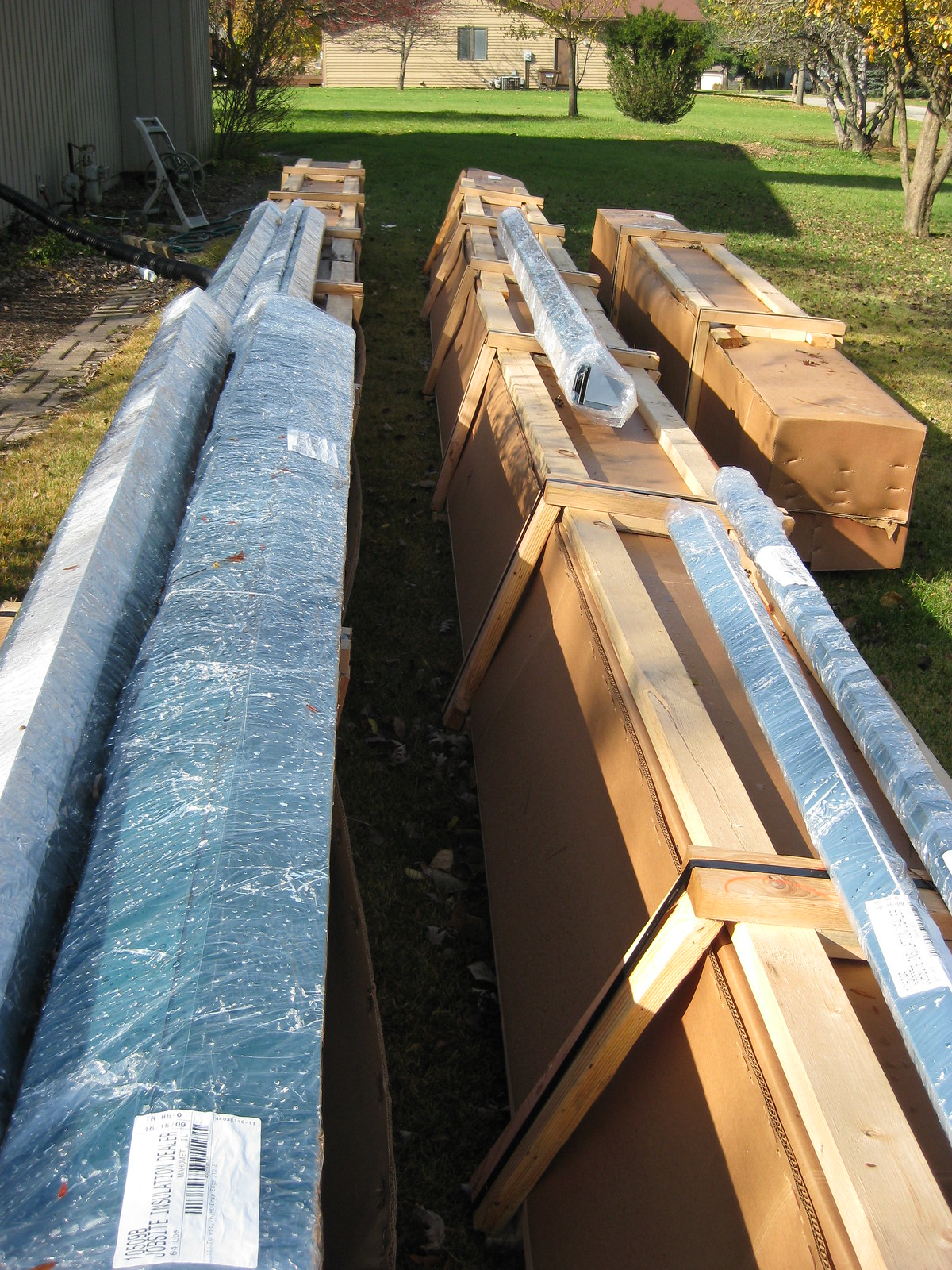The image depicts an outdoor scene in a residential neighborhood, highlighting a large collection of materials stacked next to a brown house. The materials are organized into three long rows, predominantly consisting of boxes and crates. Many of the crates feature a combination of cardboard components and wooden supportive frames, while some items are securely wrapped in clear plastic. On top of these stacks, there are L-shaped metal pieces neatly nested and also wrapped in plastic, giving them a shiny, silverish appearance. The setting is lush and green, with a vast lawn, various trees, and shrubs surrounding the area. The house in the background has tan wooden siding, a central window, and a door on the far right. Near the stacked materials, to the left, is a flower bed defined by brick or concrete pavers, along with a hose reel affixed to the side of the building. The overall scene is captured in daylight, showcasing the vibrant colors and natural elements of the environment.